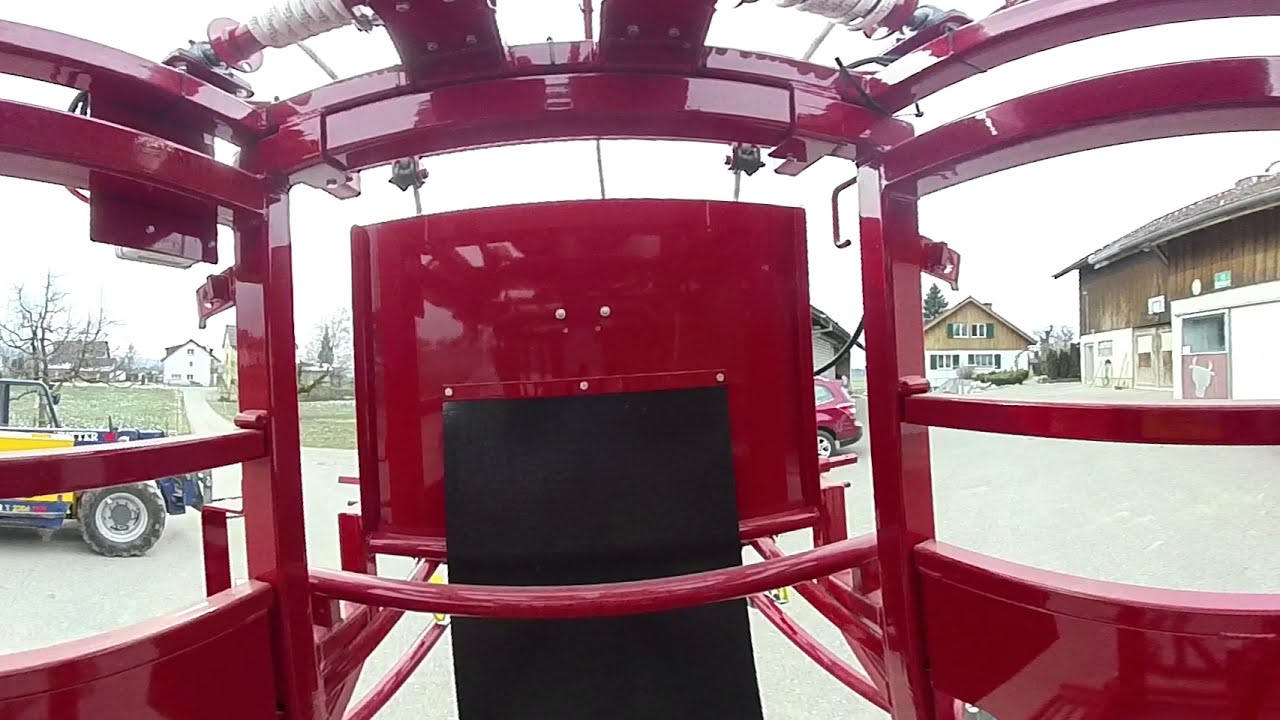This image, captured from the inside of a large piece of machinery, features an intricate metal frame predominantly colored in red. The machinery occupies the entire foreground, offering a segmented view of the surroundings through its gaps. In the center lower region, a conspicuous black rectangle aligns with the structure. Beyond the left side of the red framework, a vibrant yellow truck with large black wheels stands prominently. The right side of the image reveals two buildings—a white-bottomed structure with wooden panels and shutters at the top, resembling a barn or stable, and another brown and white house. Peeking through the metal gaps in the middle is the back end of a maroon-colored car. The background also includes a green grassy area and a leafless tree, suggesting an early spring or late autumn setting. The overcast sky adds a muted tone to the overall scene, captured from what appears to be a driveway. There is no text within the image.